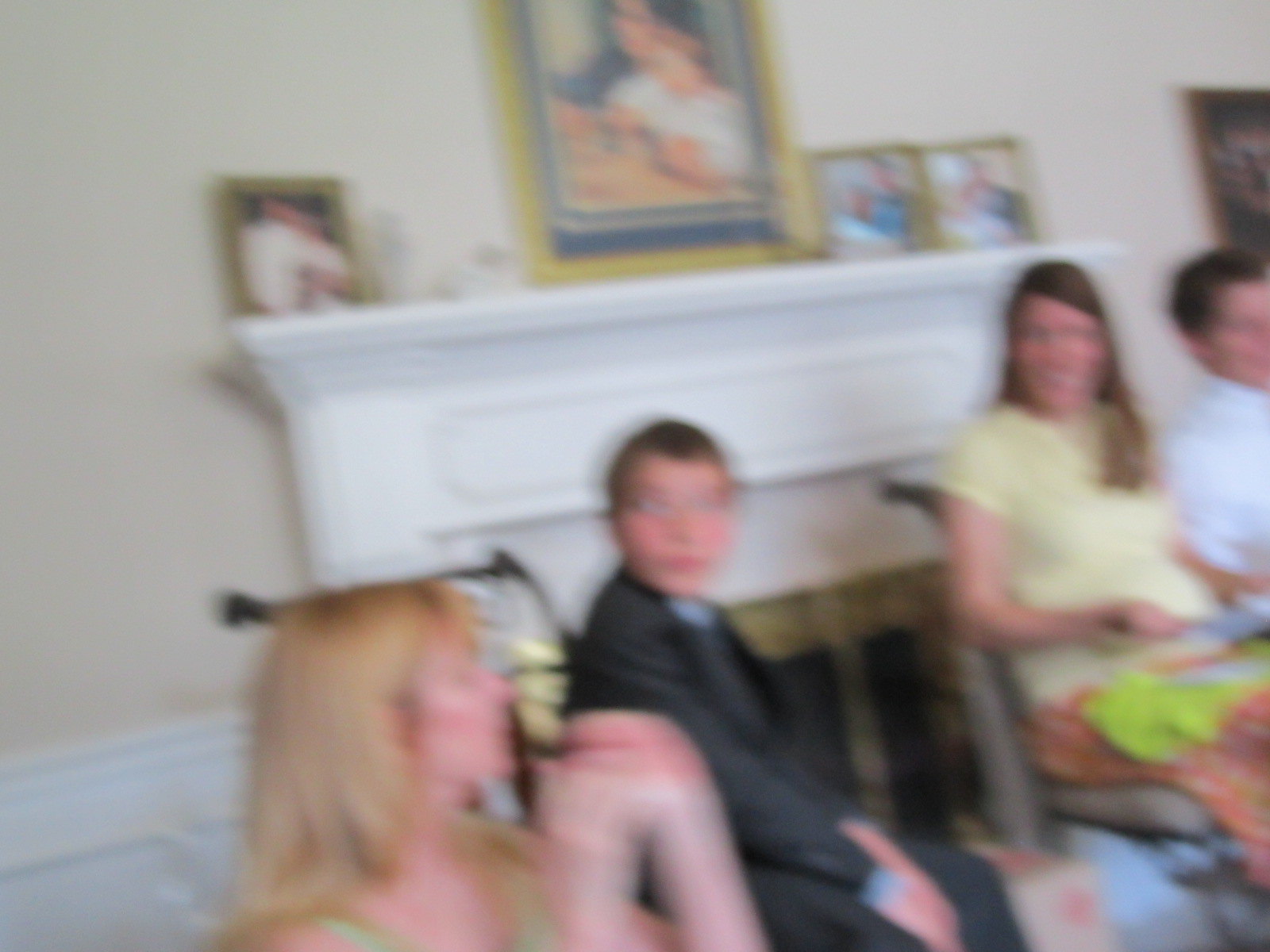A very blurry image captures a group of four individuals seated in front of a detailed fireplace. The fireplace features a gold and black covering, a large white mantle, and several gold-framed family photographs above it. At the bottom of the image is a blonde woman with noticeably red skin, possibly wearing a green tank top. She is seated next to a man in a black long-sleeved shirt, while on his other side, there is a woman with long brown hair in a yellow shirt and possibly a pink skirt or dress, holding something lime green in her lap. To the right of her, a man in a white long-sleeved shirt with a collar is seated, and he appears to be a younger boy with short brown hair. Despite the overall blur, the scene suggests a cozy, intimate setting, perhaps a family gathering.